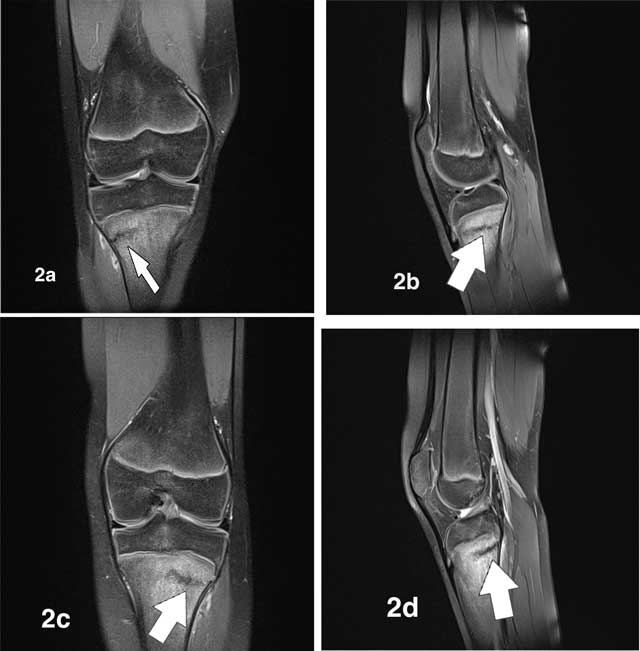The image comprises four black and white x-rays of a non-human joint, possibly from an animal, with clear indications of a crack or fracture. The x-rays are labeled 2A, 2B, 2C, and 2D, each presenting the joint from different angles: front, left side, back, and another side angle. Each x-ray features a white arrow pointing to the problematic area of the joint, likely the crack or fracture, which is visible in all images. These arrows, along with the labels against a black background, make the issue stand out prominently. The joint in question could resemble either a knee or an elbow, as they show two bones meeting, with the crack highlighted clearly in all views.